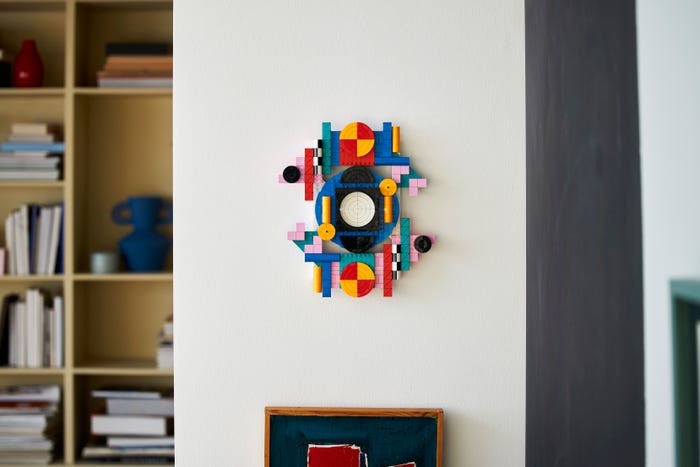A detailed photograph in a landscape layout captures an indoor scene where a white wall, centrally positioned, features an intricate art piece. This artwork, resembling a structured mosaic, incorporates various geometric shapes such as squares, rectangles, and circles. Dominant colors in the piece include blue, green, pink, red, yellow, white, and black. At the art's core, a black circle is flanked by a red and yellow circle above and below it, all surrounded by a series of golden keys. The outer edges of the piece comprise teal and pink rectangles.

Below this striking artwork is a partially visible brown picture frame with a black background and red details, contributing further to the room's aesthetic. 

To the left, a built-in wooden bookshelf stands, filled with numerous books. The topmost shelf holds a red vase, while a blue vase is placed on the second row down on the right-hand side. The right section of the photo reveals another segment of a wall, appearing in charcoal gray, just next to a brief view of a white section and a possibly green part of another shelf. The overall image is bright and clear, with exceptional lighting that illuminates all elements in the scene.